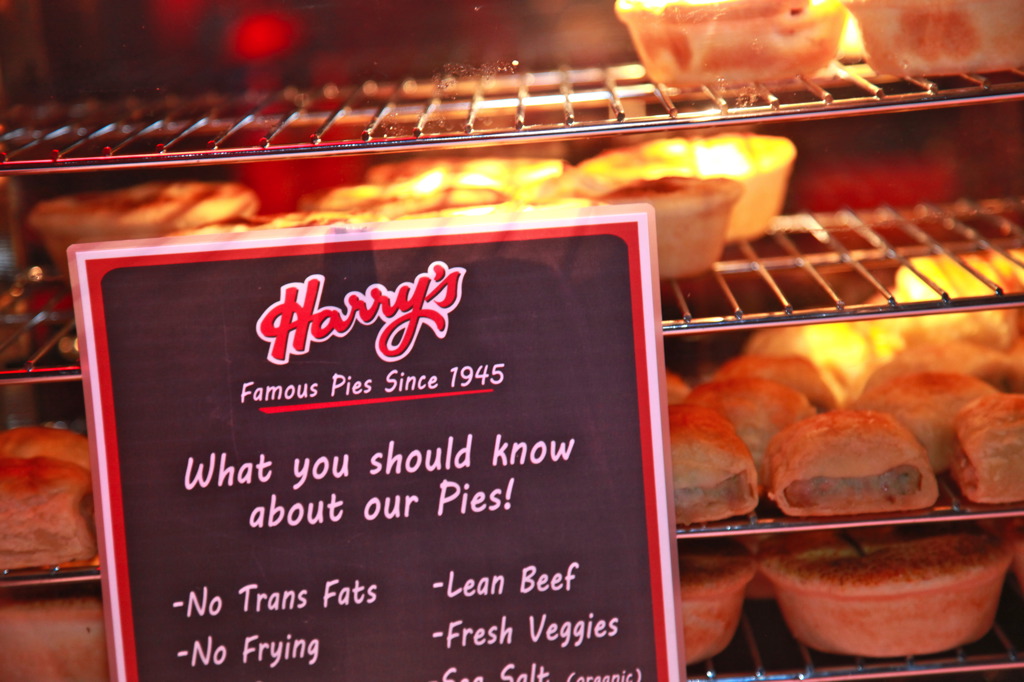This photograph shows a bakery window display case, viewed through a slight glass reflection. The display features rows of metal cooling racks, each filled with various types of pies. The pies are backlit by warm orange and golden lighting, enhancing their appetizing appearance. Some pies are circular while others are oblong, and you can see the fillings in the oblong ones, suggesting they are likely meat and vegetable pot pies. Attached to the glass of the display case is a prominent black sign with a red border. The top of the sign features a red logo with a white border, written in cursive as "Harry's." Below the logo, in white text, the sign proudly states "Famous pies since 1945." It continues with a list of pie attributes: "What you should know about our pies - No trans fats, no frying, lean beef, fresh veggies, sea salt." The rich details and the description of the sign provide a clear indication of the bakery's dedication to quality and tradition.